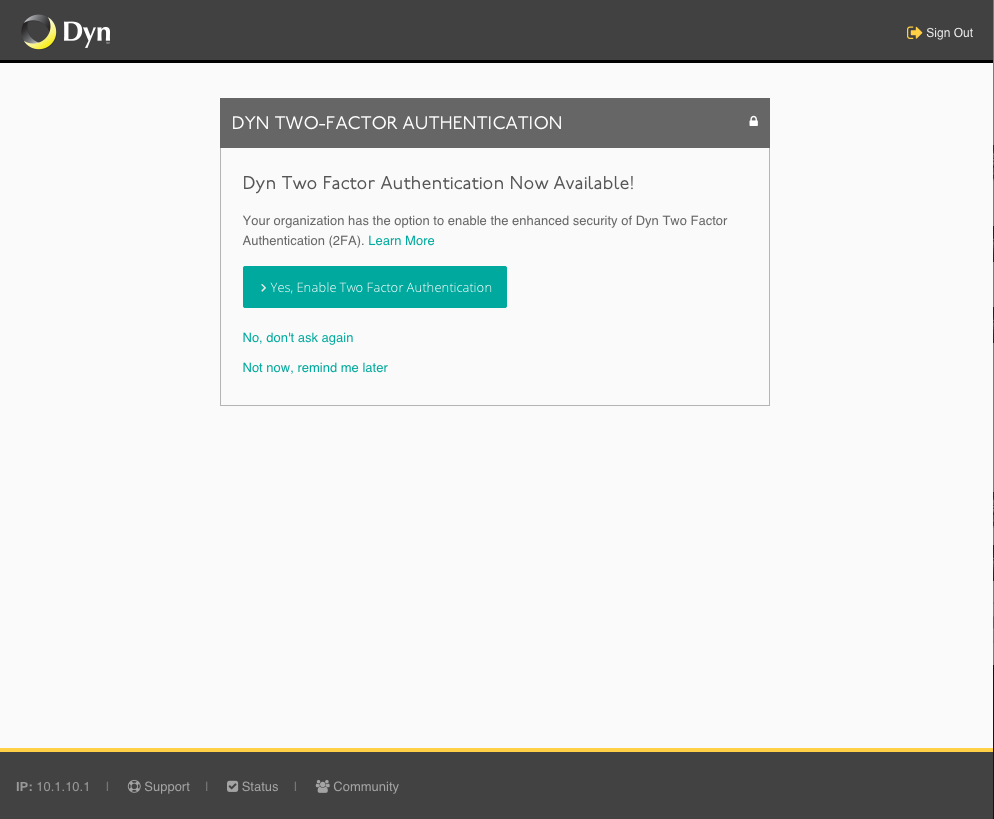Screenshot from a web application displaying a DYN interface with a Two-Factor Authentication prompt.

The top and bottom of the screen feature black bands, with the bottom band having a yellow edge. Dominating the header area is a logo comprising a yellow crescent moon shape on the left and a black circle behind it, marked with the text "DYN." To the right of the logo, a small yellow button labeled "Sign Out" is visible in white text.

The body of the page has a grey background and includes a pop-up window for Two-Factor Authentication. This window features a grey header bar with the message "DYN Two-Factor Authentication" and a white padlock icon on the right. The main body of the pop-up reads: "DYN Two-Factor Authentication now available. Your organization has this option to enable the enhanced security of DYN Two-Factor Authentication (2FA)." There is a green "Learn more" link beneath this text.

Further within the pop-up are two green buttons. The top button, which says "Yes, enable Two-Factor Authentication," uses light green text that is difficult to read against its dark green background, presenting a design flaw. The bottom button offers options "No, don't ask again" or "Not now, remind me later," also in green text.

Along the bottom black band of the screen, there are barely visible icons for IP address, support, status, and community, suggesting additional navigational options or features.

Overall, the design choices, particularly the use of light green text on a dark green button, compromise readability and accessibility for users with visual impairments.